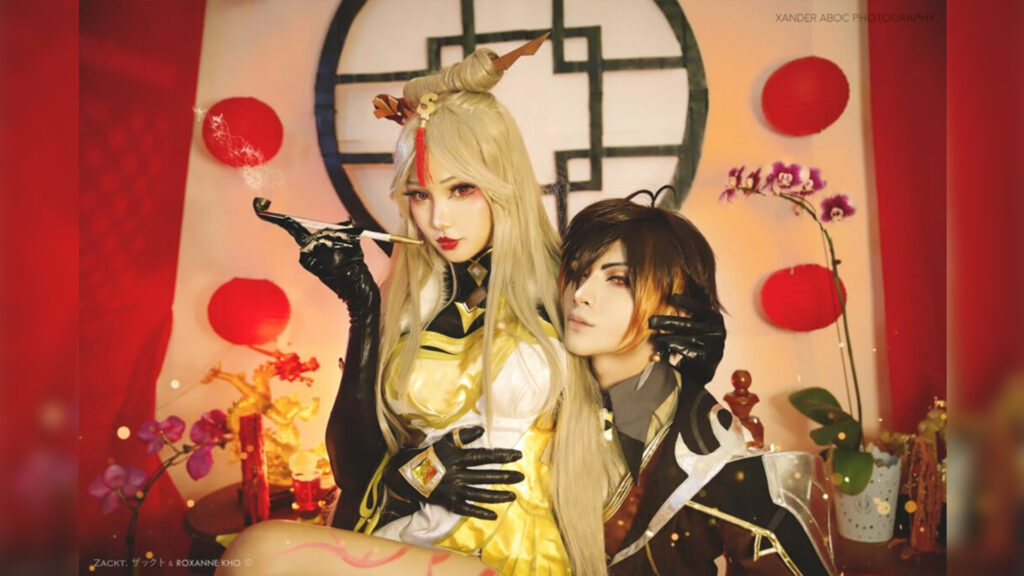The photograph captures a striking scene of a cosplay couple dressed as anime characters, both with pale complexions and heavy makeup. The woman, seated on the man's lap, has long blonde hair adorned with red tassel-like ornaments on her forehead. She is dressed in a yellow frock paired with black gloves and holds a cigarette and a pipe. The man, positioned to her right, looks mannequin-like with straight dark brown hair and is dressed in a black and brown jacket or suit, also wearing black gloves. The background includes vibrant red curtains on either side, framing a beige wall with a central circular symbol featuring four red circles. Orchid plants add a touch of nature to the scene. The bright, natural lighting enhances the clarity of the image, which bears the watermark "Zander ABOC Photography" in the top right corner, suggesting the photograph's professional provenance.